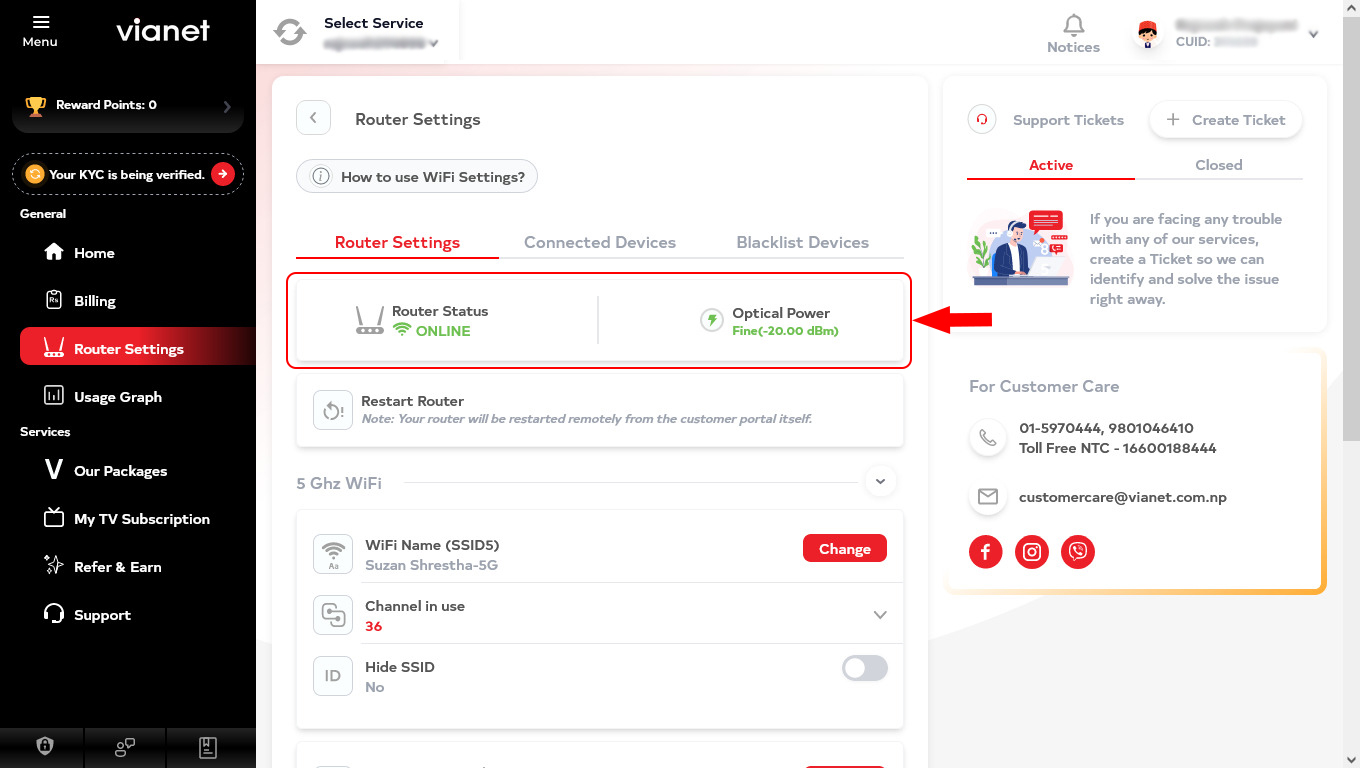**Screenshot of Vianet User Interface:**

The screenshot captures the interface of a Vianet service portal. On the left side, there's a black column with a structured menu. At the top, there is a menu title represented by three white lines labeled "Vianet." Below it, you see a trophy icon indicating "Reward Points: 0" followed by a message "Your KYC is being verified" accompanied by a red arrow.

Further down, the menu lists various sections:
- **General**
  - Home (with a home symbol)
  - Billing (with a billing symbol)
  - Router Settings (highlighted in red with a router icon)
  - Usage Graph (with a small square icon)
  - Services
    - VR Packages
    - My TV Subscription (with a TV screen symbol)
    - Refer and Earn (with a unique star icon)
    - Support (with a headphones and microphone icon)

At the bottom of the column, there are additional icons: a crest with a lock, conversation bubbles, and an image of a paper sheet.

The main area of the page is predominantly white. At the top, it starts with a section titled "Select Service" featuring two circular arrows. Below this is a pale pink line followed by "Router Settings" with a leftward pointing arrow. An oval button labeled "How to Use Your Wi-Fi Settings" is present.

Immediately below, there is a red rectangle with tabs for "Router Settings" (highlighted in red), "Connected Devices" and "Blacklist Devices" (both in gray). Below these tabs is a box showing "Router Status: Online" in green and "Optical Power: Fine."

There is a "Restart Router" button with some text beneath it. The 5GHz Wi-Fi settings section has three options: "Wi-Fi Name (SSID)" "Channel in Use," and "Hide SSID," with the "Change" button in red on the right.

In the upper right corner, there are icons for notifications - a bell and a user profile symbol. Below these, there are buttons for "Support Tickets" and "Create Tickets." The status of tickets is shown with "Active" in red and "Closed" in gray.

At the bottom of this section, an animated image shows a man at a desk with text prompting users facing service issues to create tickets for assistance. It shares customer care contact details, including a phone number, email address, and social media icons for Facebook, Instagram, and Messenger in red bubbles.